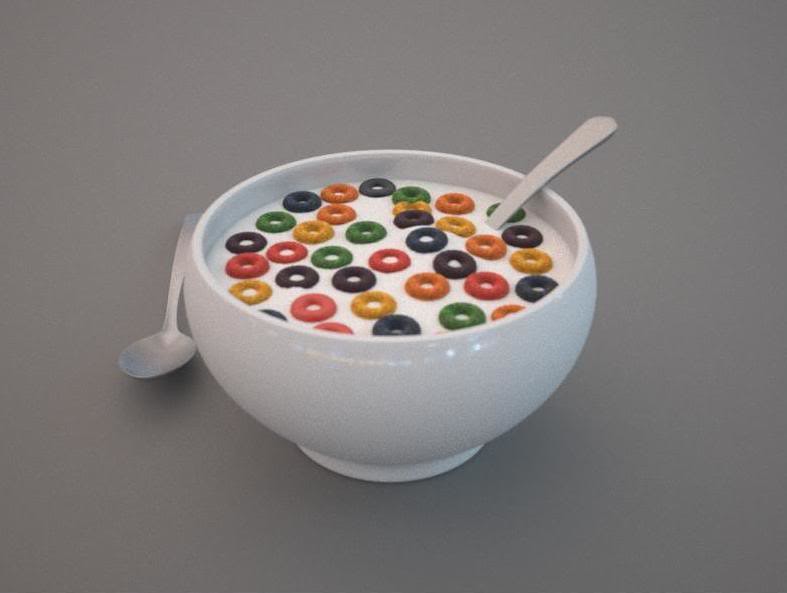The image is a close-up digital photograph of a shiny white ceramic bowl filled almost to the brim with milk, topped with a small amount of multicolored, circular cereal pieces resembling Froot Loops. The cereal pieces, arranged neatly, create a striking contrast against the white milk, highlighting colors such as yellow, orange, pink, purple, and green. Inside the bowl, a silvery metal spoon is submerged in the milk, while another identical spoon rests on the left side of the bowl, lying on the gray-colored background surface. Reflections on the bowl's surface indicate its glossy, reflective nature, suggesting it is made from a high-polish ceramic material. The overall composition gives a sense of meticulous arrangement, possibly AI-enhanced, to achieve a perfect, almost surreal appearance.